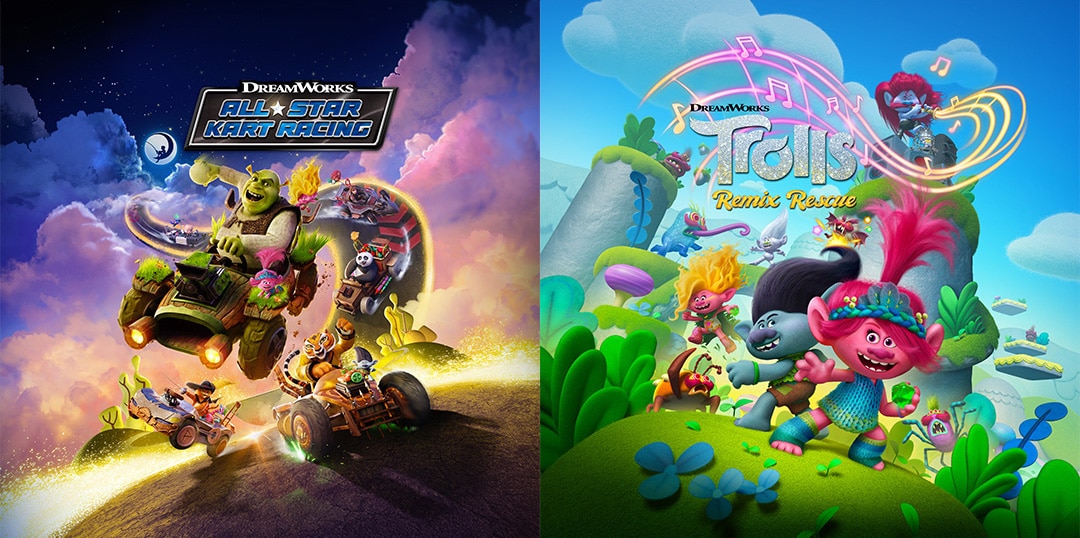The image consists of two adjacent promotional posters for DreamWorks video games. The left poster, titled "DreamWorks All-Star Kart Racing," showcases a lively kart race featuring characters from various DreamWorks films. At the center, Shrek is airborne in a wooden go-kart, accompanied by Puss in Boots and a tiger in similar karts beneath him. The background reveals Kung Fu Panda navigating the zigzagging track that ascends into a starry night sky, adorned with pink and blue clouds. Overseeing the scene is the iconic boy fishing from a crescent moon in the top-left corner.

The right poster promotes "DreamWorks Trolls Remix Rescue," depicting vibrant Trolls characters on a gently sloping, green grassy hill. Central to the image is a pink Troll with spiky pink hair, accompanied by a green-skinned Troll flaunting a black pompadour. Behind them, another Troll with voluminous blonde hair adds to the ensemble. The background features pastel-toned clouds and hills beneath a blue sky. Musical notes and lines gracefully float above the characters, emphasizing the musical theme. Both titles, "DreamWorks All-Star Kart Racing" and "DreamWorks Trolls Remix Rescue," are prominently featured in their respective images, each highlighting the colorful, whimsical nature of the games.